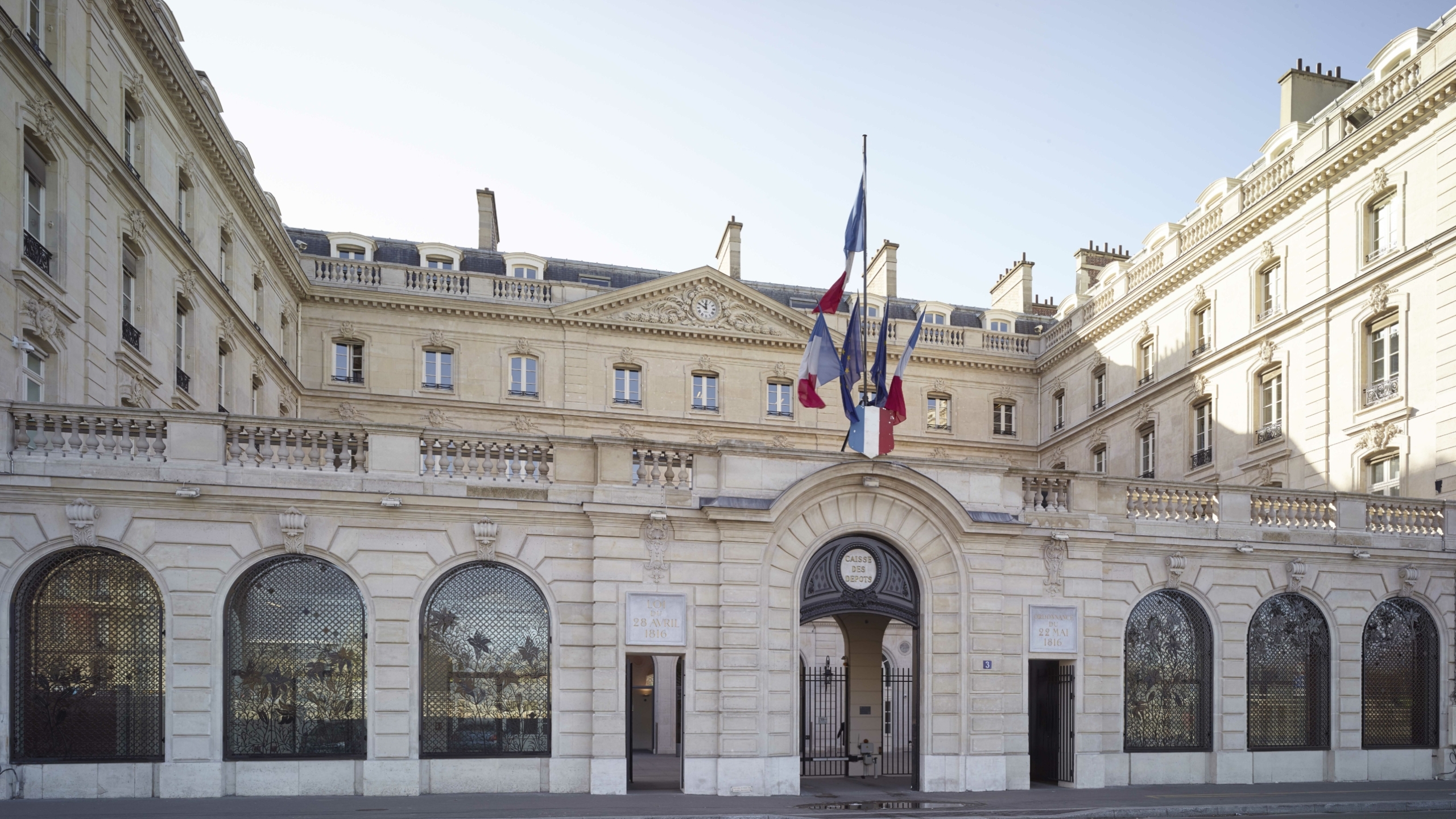The image features a large, European government building with a U-shaped layout and a light cream-colored stone façade. The front is marked by big arched windows, each adorned with black barriers or screens for protection. Dominating the entrance is an arched doorway with ornate black metal gates, flanked by two additional doors, one also gated. Above the entrance, a series of blue, white, and red flags—distinctly non-American—are displayed prominently. A plaque is visible above the doorway, though it is too small to read clearly. The building stretches up three to four stories, with the front transitioning to a slightly yellow-hued stone surface towards the back. In the center of the upper section, there is a small circular feature with a white clock and black hands, topped by an arched roof. Further back, a taller structure peaks with a blue section against a sky that fades from blue on the right to white on the left. The overall color palette of the building is predominantly white, tan, gray, and black, with the vibrant flags providing a striking contrast in the middle of the photograph.